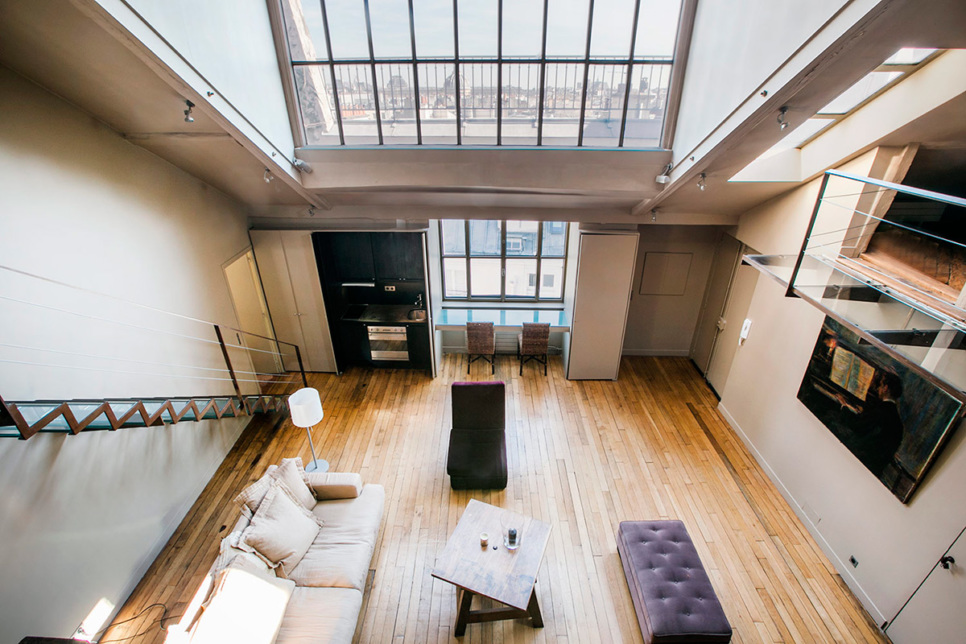The image depicts a sophisticated urban apartment viewed from above, giving a clear perspective of an open-plan living room. The room features light white hardwood flooring and a beige couch positioned to the left. Central to the room is a distinctive wooden coffee table set askew on black supports. To the right of the table is a unique purple velvet bench, adjacent to which is a black chair with a purple back. This setup is complemented by an elegant kitchenette with predominantly black cupboards located behind the sitting area. 

To the right of the kitchenette, there’s an inset blue desk flanked by two wooden chairs. Next to this workspace is a white, blank cabinet. Between the kitchenette and the cabinet, a set of window panes offers a view of an Italian cityscape, with a prominent domed roof visible in the center frame beneath a clear pale blue sky. On the left, a glass stairway with simple metal banisters and black vertical posts ascends toward the observer, blending seamlessly into the modern design of the room.

On the right side, a gray wall hosts a television beneath an overhead glass viewing area supported by black horizontal beams, under which a brown mattress in a loft area is partially visible. The sloped ceiling extends from the center upwards, enhancing the spacious feel of the apartment, while large windows flood the room with natural light and frame a picturesque urban landscape.